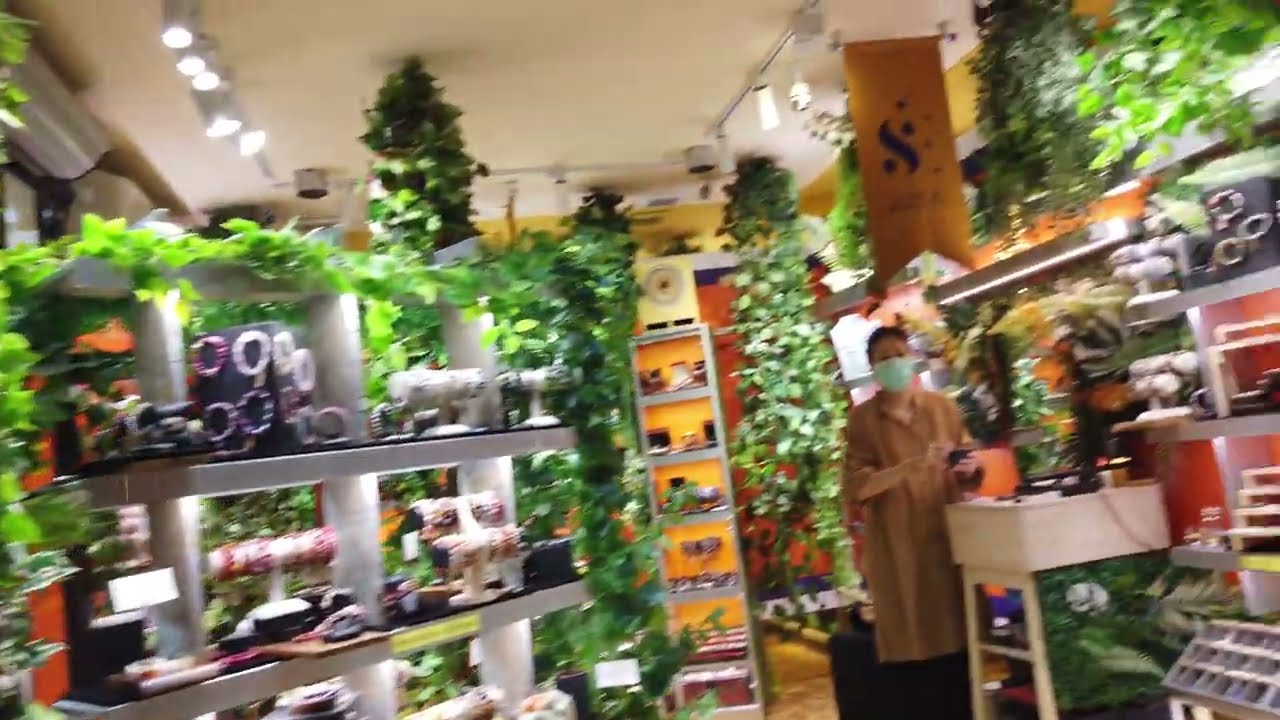The image depicts the inside of a jewelry store, albeit slightly blurry and out of focus. The store is filled with an abundance of greenery, with light green plants and vines cascading from the ceiling and adorning the shelving units. On the left side of the image stands a large, multi-level white display case, showcasing various pieces of jewelry including necklaces, bracelets, and earrings. These display units are surrounded by lush green leaves and vines, enhancing the natural decor of the store.

To the right, a woman wearing a blue face mask and a long, medium-brown shirt stands near a small beige wooden desk. Directly above her hangs a distinctive yellow banner with a black 'S' and some decorative dots and lines ending in an arrow shape. The store’s ceiling features lighting that illuminates the merchandise below. The warm orange walls add a cozy feel to the environment, contrasting with the greenery and enhancing the overall aesthetic of the store.